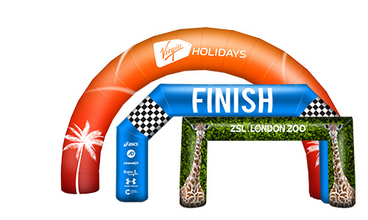The image features a series of inflatable finish lines set against a white backdrop, showcasing different designs and color schemes. The foremost finish line is green, rectangular in shape, and the shortest. It is adorned with a giraffe print on both sides, with the giraffes' necks extending upwards amidst a leafy green background. Across the top, it reads "ZSL London 200." Placed behind it is a blue arch with an octagonal shape, characterized by a checkered flag pattern on the sections connecting the pillars. The word "Finished" is prominently displayed in white across the top. Furthest back, a semi-circular orange arch looms tallest. It features white palm tree patterns at the base, and the text "Virgin Holidays" in white and orange spans the top.